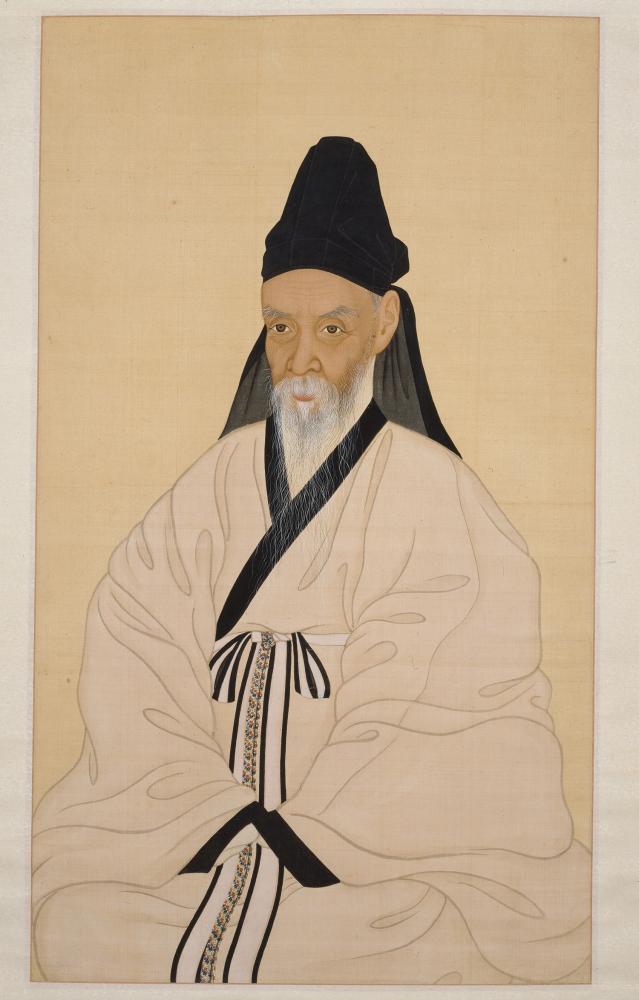This is an artistic painting on a beige canvas, depicting an elderly Asian man, possibly of Japanese origin, with olive-complected skin. The man has bushy gray eyebrows, brown eyes, and a long, scraggly white beard with gray accents that extends up the sides of his face. His mustache and goatee are similarly wispy. He wears a distinctive black head covering that peaks to a rounded top and drapes down behind his head.

The man is garbed in a voluminous beige ceremonial robe that conceals his hands and legs, suggesting he is seated or kneeling. The robe, richly detailed, features black trim at the neck and wrists, and a white belt with alternating black and white stripes, tied around his waist. The robe also has white stripes running down the center, connected to the belt, and a delicate embroidery between these stripes. The background is a light brown color with a light gray outer barrier, enhancing the painting’s antiquated and dignified appearance.